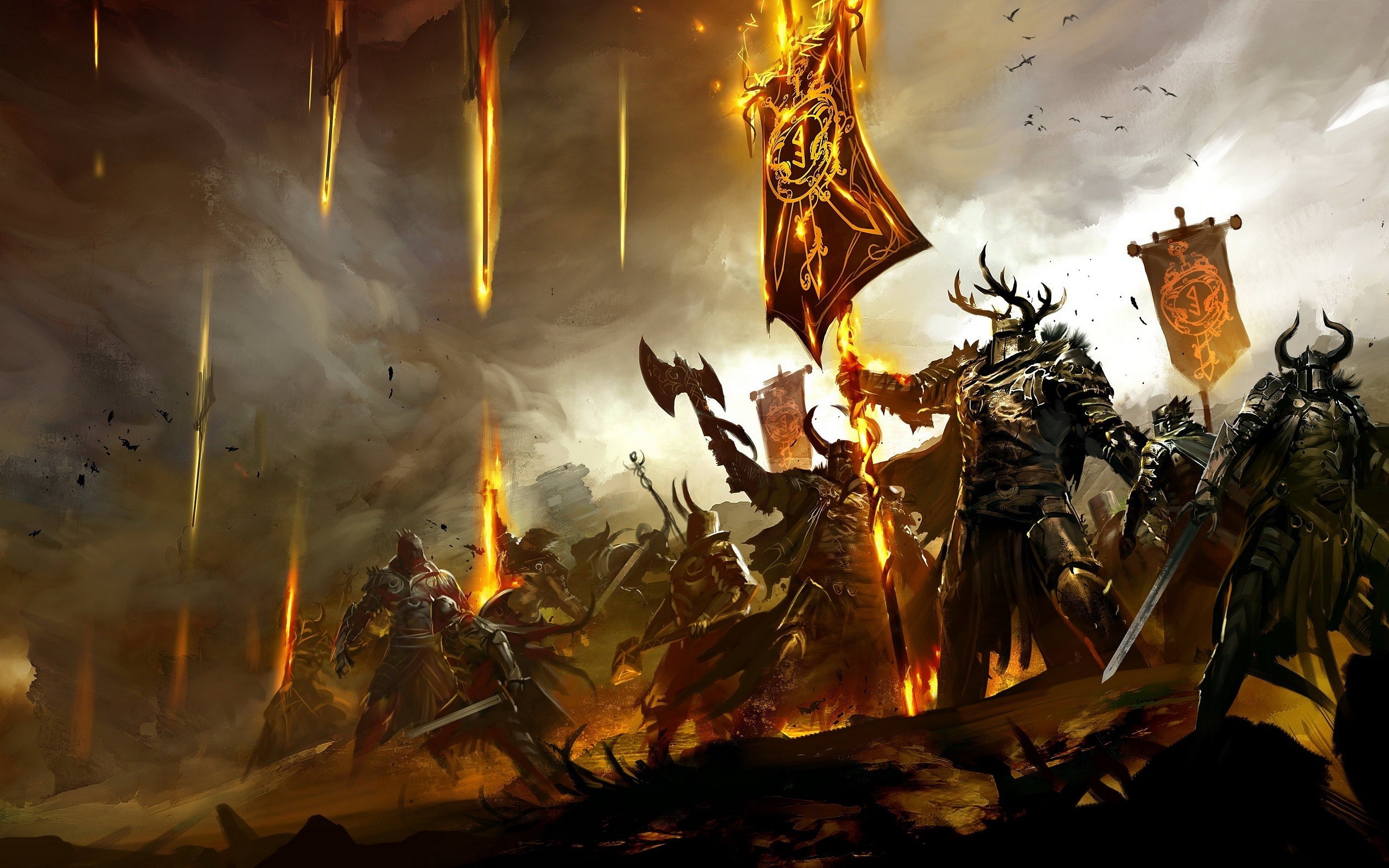The image depicts a dramatic, computer-generated medieval battle scene, likely from an animated movie or a video game. Warriors clad in silver body armor, some adorned with helmets featuring fearsome bull horns or intricate deer antlers, charge forward with an array of weapons including swords and axes. The atmosphere is grim and dark, with swirling black smoke and apocalyptic fire raining from the sky, casting an ominous glow. At the forefront, a key figure stands on a hill to the right, bathed in light. He wears a distinctive helmet with elaborate antlers and holds a flag that is ablaze, its red and black emblem nearly obscured by flames. Similar flags, some also on fire, illuminate the scene with a powerful orange hue, suggesting a magical significance. Behind him, additional warriors bearing swords, axes, and staffs advance into the fray, while in the distance, faint sunlight breaks through the oppressive clouds, adding a glimmer of hope amidst the chaos.